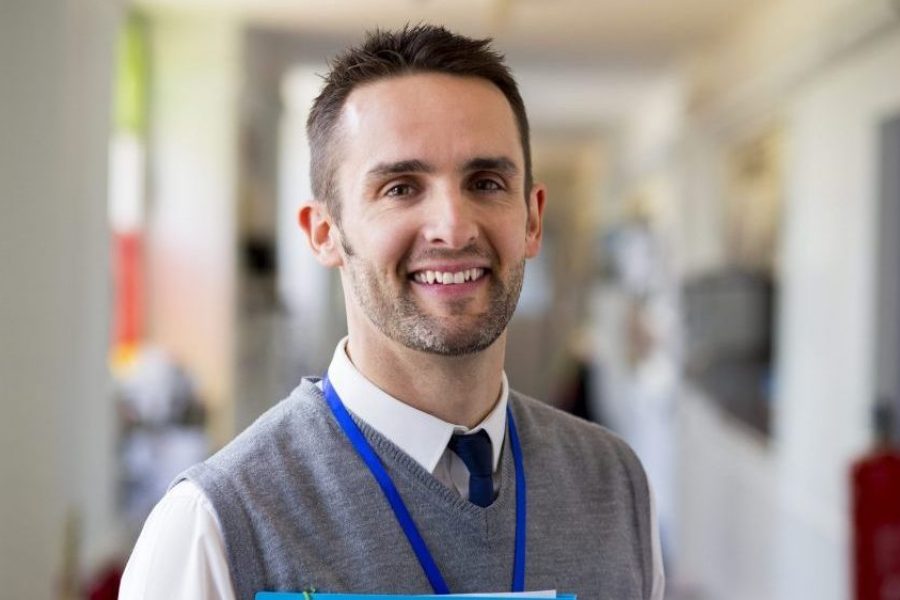The image features a professionally dressed young Caucasian man with short brown hair and brown eyes, smiling directly at the camera. He sports a 5 o'clock shadow and is depicted from his shoulders up, positioned with his right shoulder slightly closer to the camera. He is wearing a white dress shirt beneath a grey sweater vest, complemented by a blue tie and a blue lanyard around his neck, possibly holding an ID tag or similar accessory. His left hand holds a barely visible turquoise folder. The background, though blurred, suggests an indoor setting, likely an office or academic institution, with off-white walls, various cut-out windows, and doorways, lit by natural sunlight streaming in.